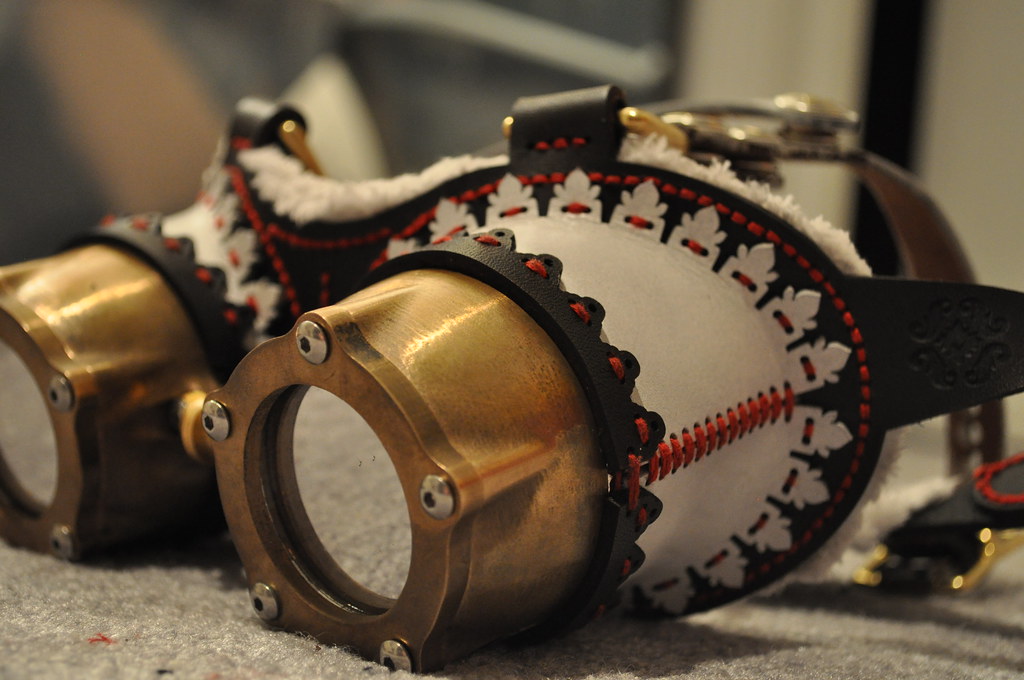This detailed and descriptive caption amalgamates elements from each provided description into a coherent single paragraph:

In a full-color, close-up photograph, a pair of homemade steampunk goggles is showcased, set upon a short, gray carpet. The image, likely taken indoors under artificial light, reveals the intricate details of the goggles. The lens frames are crafted from bronze, adorned with multiple silver screws that secure the reflective silver lenses in place. Surrounding the frames are black and white leather decorations, intricately held together with red stitching. On top of the goggles, rings are threaded through additional leather loops, while brown leather straps, designed to wrap around the head, feature a functional buckle for adjustment. Soft leather padding with fur lining ensures comfort against the face. The background of the image remains out of focus, drawing attention to the meticulous craftsmanship of the steampunk goggles.